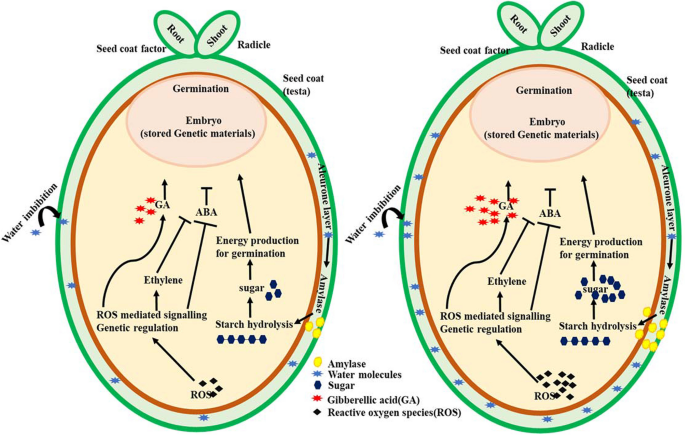This detailed digital illustration represents a biological germination pathway in plant embryos. The image is split into two sections, each depicting a germinating seed embryo with a green outer oval labeled as the seed coat. Inside each seed coat, there is a yellow internal section representing the embryo. Both embryos showcase key components involved in germination: root, shoot, seed coat factor, and radicle.

The illustration is filled with various small objects and connections, highlighting essential elements and processes. Yellow dots indicate the enzyme amylase, blue splashes represent water molecules, blue hexagons denote sugar, red splashes mark gibberellic acid (GA), and black diamonds signify reactive oxygen species (ROS). Lines and pathways connect these elements, illustrating ROS-mediated signaling, genetic regulation, ethylene, GA, and ABA’s role in energy production for germination. The embryos share common features, though the left image appears to have more detail compared to the right. The text and labels in the image are primarily black, providing clear and informative annotations. This comprehensive illustration effectively explains the complex biochemical interactions involved in seed germination.